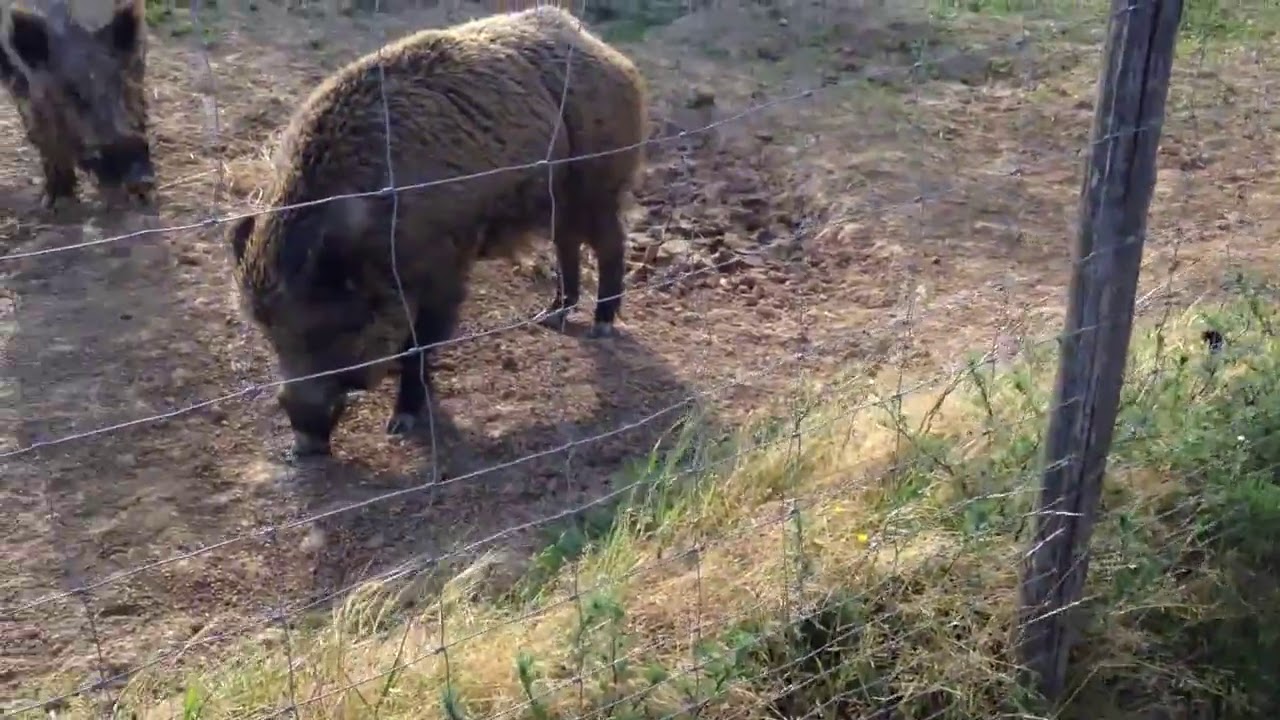This photograph shows two large, brown, and furry pigs, possibly boars or warthogs, enclosed within a wired fence made up of square grids. The pigs, bearing thick winter coats, stand on a bare, dirt-covered ground with noticeable ruts. Their fur exhibits a mix of brown and darker shades, especially on their snouts, inner ears, and just above their hooves. The sparse green and brown grass along the fence contrasts with the predominantly dirt-filled enclosure. The silver fencing, attached to weather-beaten dark silver posts, separates the enclosure from a slightly blurry background. The sun casts distinct shadows of the pigs, enhancing the natural lighting of the scene and highlighting the varied textures and hues of both the pigs and their surroundings.